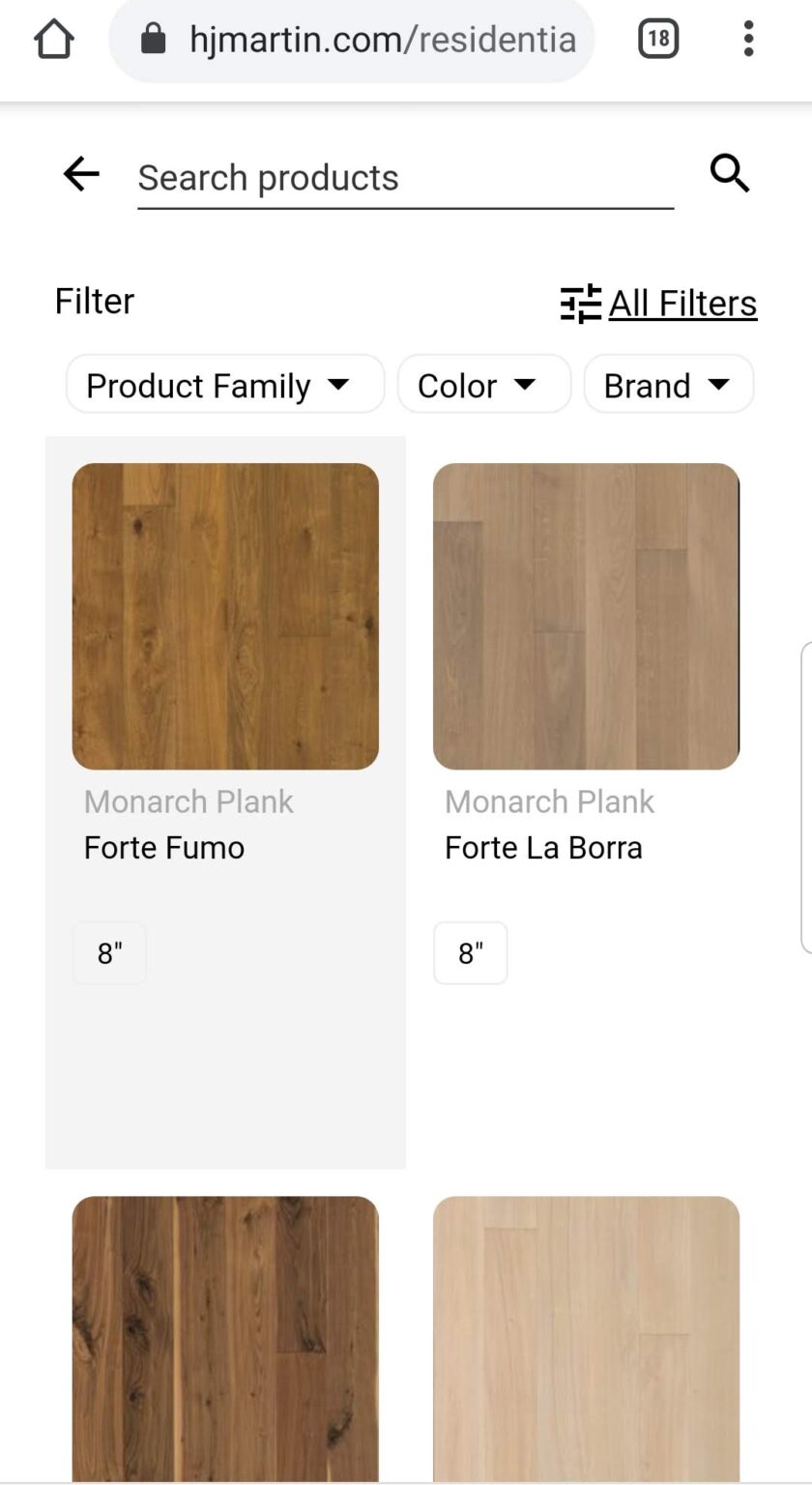This mobile screenshot captures the user interface of an online flooring product page from hjmartin.com, specifically under the residential section. At the uppermost portion of the image, the address bar is visible with a home icon, followed by the URL "hjmartin.com residential." To the right of the address bar, there's a box indicating the number 18, likely denoting active tabs, and three vertical dots symbolizing additional options.

Beneath the address bar is a navigation line featuring a left-pointing arrow labeled "Search Products" accompanied by a magnifying glass icon on the right. Directly below this is a filter section with options labeled "Filter" on the left and "All Filters" on the right, followed by filter buttons for "Product," "Family," "Color," and "Brand," each with a downward-pointing arrow indicating expandable menus.

The central and lower portions of the image display samples of wooden flooring. On the left side, there's a sample labeled "Monarch Plank Forte Fumo," identified as being 8 inches wide. Next to it, on the right, is another sample named "Monarch Plank Fort La Bora," also 8 inches wide. These names likely reference the specific colors or styles of the wood.

The bottom section shows two more wood samples without any labels: a darker wood on the left and a lighter wood on the right. Additionally, towards the right center of the image, a thin gray vertical line suggests the presence of another plank or the edge of one of the displayed samples. The background of the screenshot is predominantly white, enhancing the visibility of the text and wood samples.